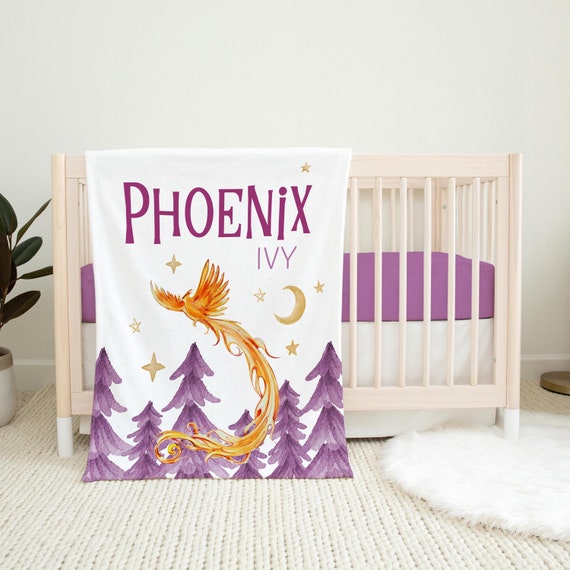This well-lit nursery features an ivory-colored wooden crib with closely spaced slats, ensuring safety for the baby. The crib, placed against a pristine white wall, houses a purple mattress resting on a white base. Enhancing the cozy ambiance, a white furry throw rug adorns the cream-colored carpet on the bottom right-hand corner. To the center left, a vibrant green plant adds a touch of nature to the room. Draped over the side of the crib is a decorative banner that reads "Phoenix Ivy" in purple letters. The banner showcases a stunning red and orange phoenix bird soaring with its wings spread wide, with purple trees in the background, and a motif of stars and a moon, tying the nursery's color theme together. The photo likely serves as a product image for a baby furniture company, offering a glimpse into a stylish and carefully curated nursery setup.